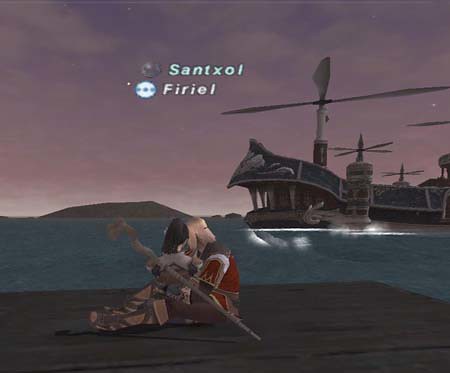The screenshot captures an atmospheric scene from a video game, with a vibrant purple sky stretching across the background. Framing the horizon are majestic mountains silhouetted against the twilight, and in the foreground, a calm body of water, either a lake or a river, reflects the waning light. On the right-hand side of the water floats a large boat, notable for its helicopter-like propellers atop it, moving toward the left side of the image.

In the immediate foreground, a wooden dock extends into the scene, with a lone character kneeling down upon it. The character, dressed in knee-high boots, a red shirt, and brown pants, appears to be holding another person protectively. Beside them rests a long staff or scepter, hinting at some form of mystical or leadership role. The character's black hair is clearly visible, suggesting a shadowy profile against the natural palette of the background. 

Interspersed in the scene are two prominent text labels: "S-A-N-T-X-O-L" positioned centrally, with "F-I-R-I-E-L" situated below it. Each word is encased in its own distinctive design, adding an element of intrigue and context to the game's world.